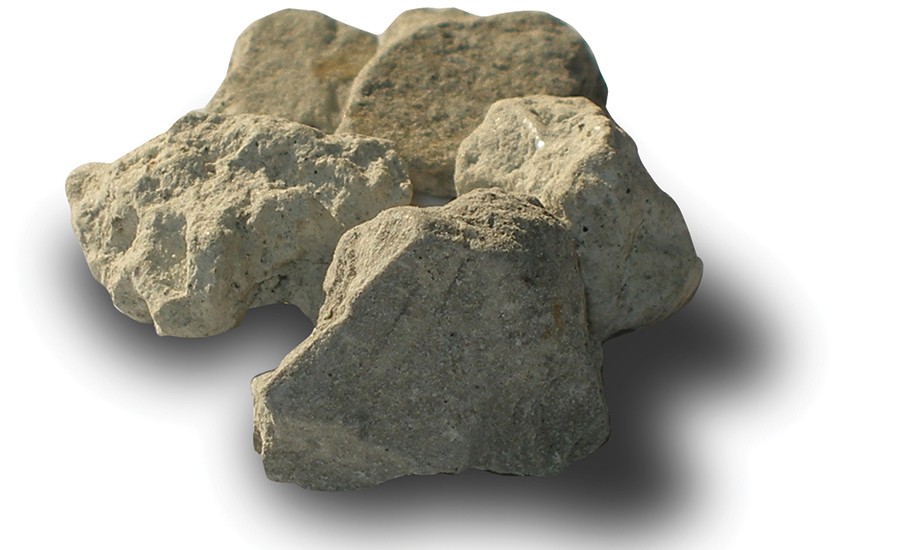The image depicts a meticulously arranged cluster of five gray rocks, striking in their varied textures and forms. Set against a stark white background, the rocks range in color from dark to light gray, interspersed with streaks and darker dots that lend them an uncanny, almost artificial appearance. The rocks vary in texture; one prominently features divots and ridges that create a rough, uneven surface, while the others are noticeably smoother. Despite this, all the rocks share a rough texture typical of gravel or roadside stones. The right-hand side of the image falls into shadow, suggesting bright lighting from the left. Each rock is distinct yet positioned to touch the others, creating a cohesive and detailed visual display that highlights their individuality and collective arrangement.